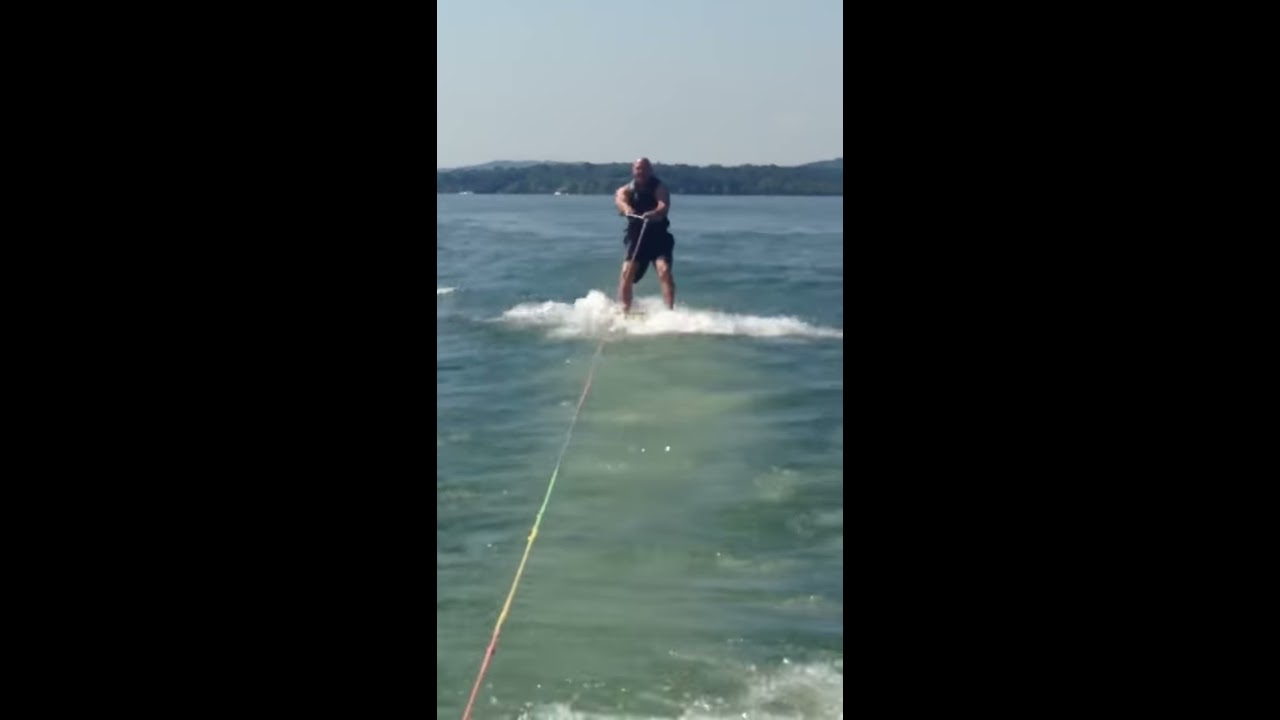The image captures a bald man, possibly a white male, engaging in water skiing while clad in black swim trunks and a black life vest. He is positioned far into the distance on the water's surface, gripping a handle attached to a long, rainbow-colored cord. The water around him is frothy and white beneath his feet, indicating movement and speed. The surrounding water is a bluish-green shade, while the sky above is clear and pale blue, taking up a quarter of the image. In the background, there is a slightly elevated, hilly landscape dense with green foliage. The vertically oriented photo is bordered on both sides by thick rectangular regions, and the horizon features a distant, tree-lined shore.